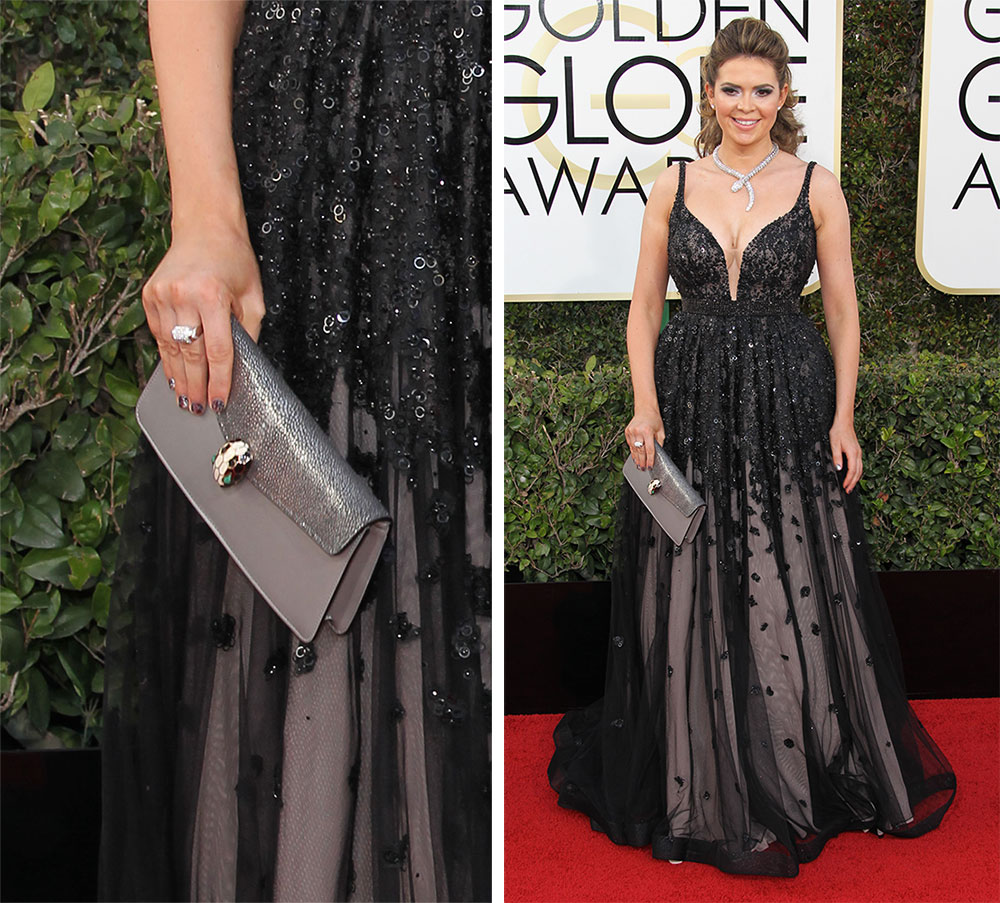This collage features two images of a female celebrity attending the Golden Globe Awards. On the right, she is captured on the red carpet in an elegant, sleeveless black sparkly gown, adorned with a striking silver snake-like necklace and a shiny ring on her right hand. Her formal hairstyle and makeup add to her sophisticated look as she stands before a sign that reads "Golden Globe Awards," against a backdrop of neatly trimmed foliage in black containers. The image on the left offers a close-up of her accessories, focusing on her gray purse with a sequin flap and an emerald-accented, insect-like clasp. This detailed perspective highlights her coordinated accessories, enhancing the overall elegance she exudes at the prestigious event.